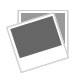The image depicts a disturbingly eerie figure, seemingly a mannequin, clad in a seemingly typical black zip-up jacket. The most unnerving aspect is the mask it wears, an unsettling contraption that combines elements from various sources of horror. The mask appears to be fashioned from a mix of sackcloth and leather, creating a patchwork effect. Its beige and skin-colored sections are held together with metallic clips, staples, and rope, mimicking scars and giving the visage a grotesque stitched-together appearance. The eyes are covered with rope in the shape of X's, with some details suggesting the eyes are eerily open underneath. The mask also features prominent lacing at the top, as if trying to keep the skull from splitting apart. Additionally, weird stitching spans the cheeks and mouth, intensifying the overall macabre look. A shadow looms behind the figure on the white wall, adding to the creepy ambiance of the photograph.